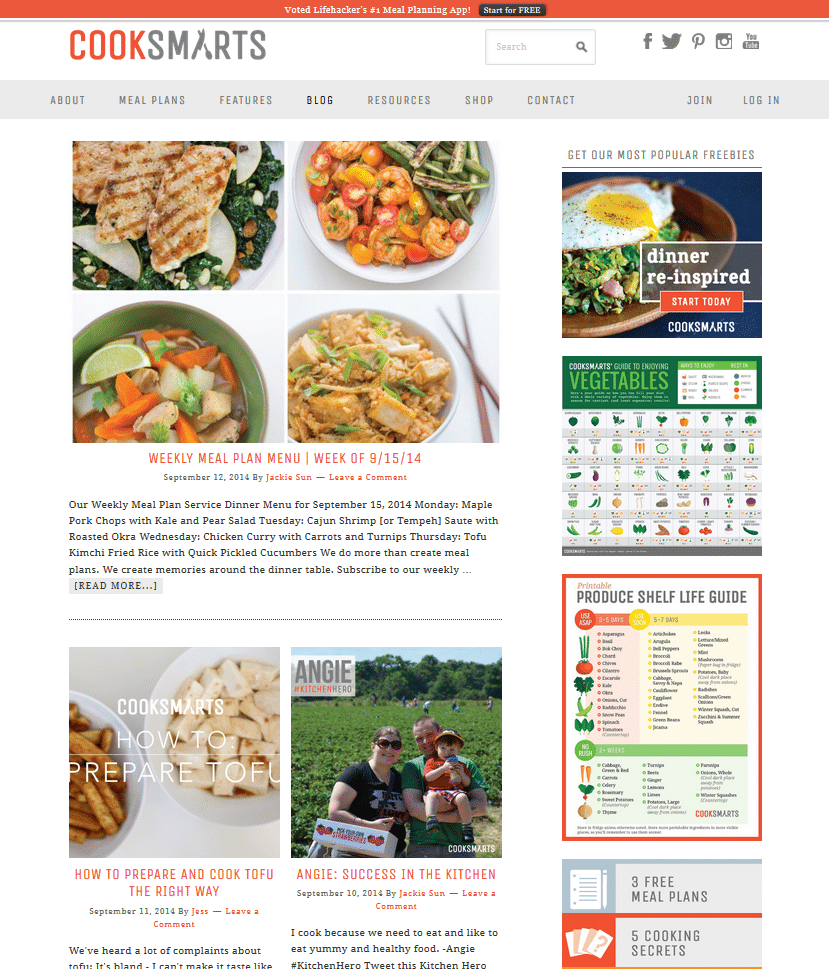This screenshot captures a web page from the website CookSmarts. At the top of the page, a thin orange banner stretches across, providing a vibrant accent to the site’s design. In the upper left corner, the CookSmarts logo is displayed in orange and gray font, adjacent to a white section. Next to the logo is a search box, accompanied by five social media icons that provide easy access to various platforms.

Below the banner, a menu bar features navigational links reading from left to right: Meal Plans, Features, Blog, Resources, Shop, Contact, Join, and Login. To the right of the main content area, a vertical column houses four advertisements and text boxes, displaying a mix of promotional content.

The primary area of the webpage, situated at the upper left, showcases a section with four appetizing photographs of healthy meals. Directly beneath this visual section, the text "Weekly Meal Plan Menu, week of 9-15-14" is displayed, followed by a detailed meal description.

Below this meal plan section, the page features two separate article teasers, each with an accompanying image. The first article is titled "How to Prepare and Cook Tofu the Right Way," while the second highlights "Angie's Success in the Kitchen."

In the right-hand column, a prominent heading titled "Get Our Most Popular Freebies" draws attention. This section contains three boxes. The top box features an image of an egg served over a dish with the caption "Dinner Reinspired." The second box displays a colorful chart of vegetables. The third box provides a "Produce Shelf Life Guide." At the very bottom, two tabs offer additional resources: "3 Free Meal Plans" and "5 Cooking Secrets," completing the rich array of content available on the CookSmarts website.